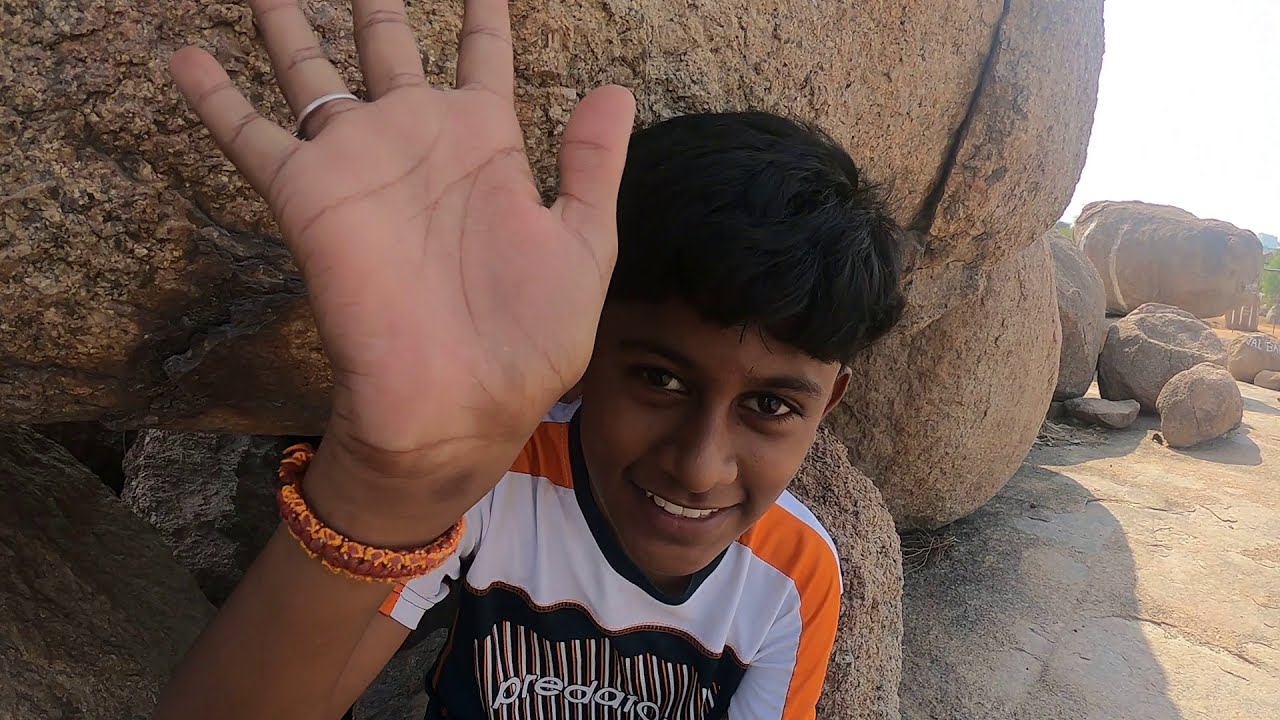In the image, a teenage boy, likely of Indian descent, is positioned centrally, smiling and looking directly at the camera. He has very dark hair and dark skin. His right hand is raised prominently towards the camera, featuring a silver ring on his ring finger and a red-orange-yellow bracelet on his wrist. He wears a white shirt with an orange stripe along the shoulders transitioning to a black area with the partially visible text "P-R-E-D-A". The boy is seated against a large tan-brown rock formation, suggesting he is in a rocky, possibly beach-like or national park setting. The background reveals other similar rock structures, a clear light blue sky, and some distant green trees. The daylight setting is evident from the sunlight casting shadows, with the sun positioned to the left.